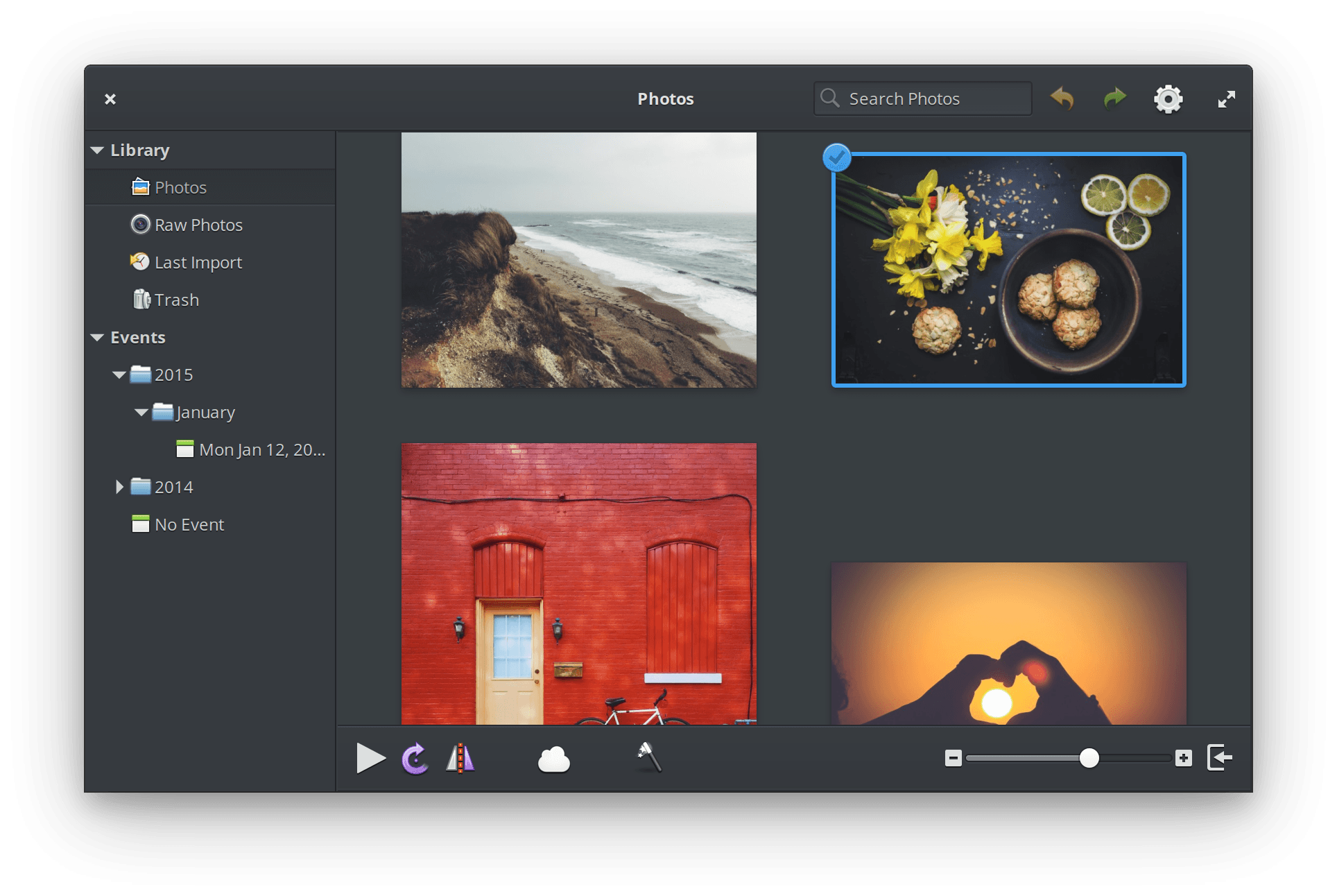The image displays an online photo application interface. At the top, the application is labeled as "Photos." On the right side of the interface, a search bar reads "Search Photos." There are various interactive icons present: a green right-pointing arrow, an orange left-pointing arrow, a gear icon, a diagonal two-arrow icon, and a left-pointing "X" icon.

On the left side, there is a navigation panel titled "Library," distinguished by a downward-facing triangle. Within the Library section, there are four subsections: "Photos," "Raw Photos," "Last Imports," and "Trash." Below the Library is a section called "Events," where several files are organized. The first file is a photo icon labeled "2015," followed by a file icon from "January," which has some of the information blocked. Further down is the date, "Monday, January 12, 2000," and below that, a file labeled "2014."